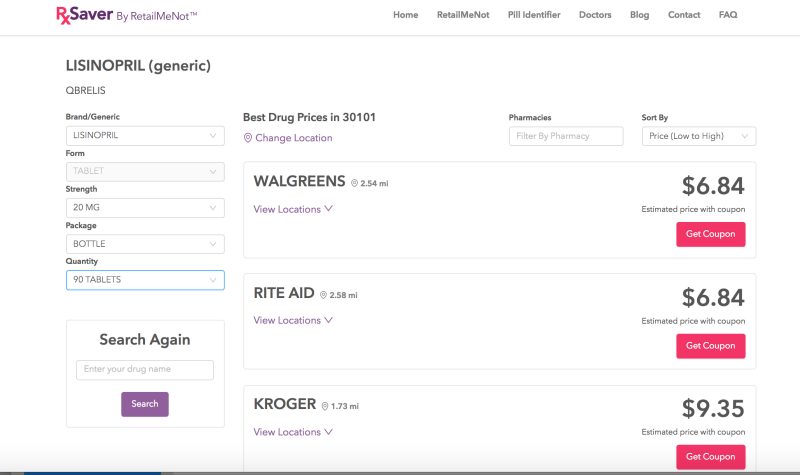**Website Screenshot Description:**

The screenshot captures a webpage prominently featuring a hot pink "RX" logo at the top left corner, with the "R" and the right leg forming the "X." Following this, the text transitions into "savor" written in a purple font, accompanied by smaller purple letters stating "buy retail, me not."

At the center-top, spanning horizontally in gray letters, the navigation menu lists multiple categories: Home, RetailMeNot, Pill Identifier, Doctors, Blog, Contact, and FAQ.

On the left side of the page, in all capital letters, the name "LISINOPRIL" appears, followed by "(generic)" in lowercase. Below it, there's a label, though the word immediately underneath is unreadable. It continues with "brand/generic," reflecting LISINOPRIL in a similar format. The page details include various drop-down options: "Form" (Tablet), "Strength" (20 milligrams), "Package" (Bottle), and "Quantity" (90 tablets). These are followed by a black search box labelled "Search Again" and a prominent purple rectangular "Search" button in white text.

To the middle of the page, it states "Best drug prices in 30101" (a ZIP code), with an option to "change location" highlighted in purple underneath.

On the right, the "Pharmacies" section includes sortable options for prices (from low to high). It lists three drugstores: Walgreens, Rite Aid, and Kroger. Each entry provides a pull-down menu to view specific locations, highlighted in purple. Prices are displayed on the right, with Walgreens and Rite Aid both at $6.84, and Kroger at $9.35, each followed by "estimated price with coupon." Beneath each price, there is a red horizontal button labelled "Get Coupon" in white text.